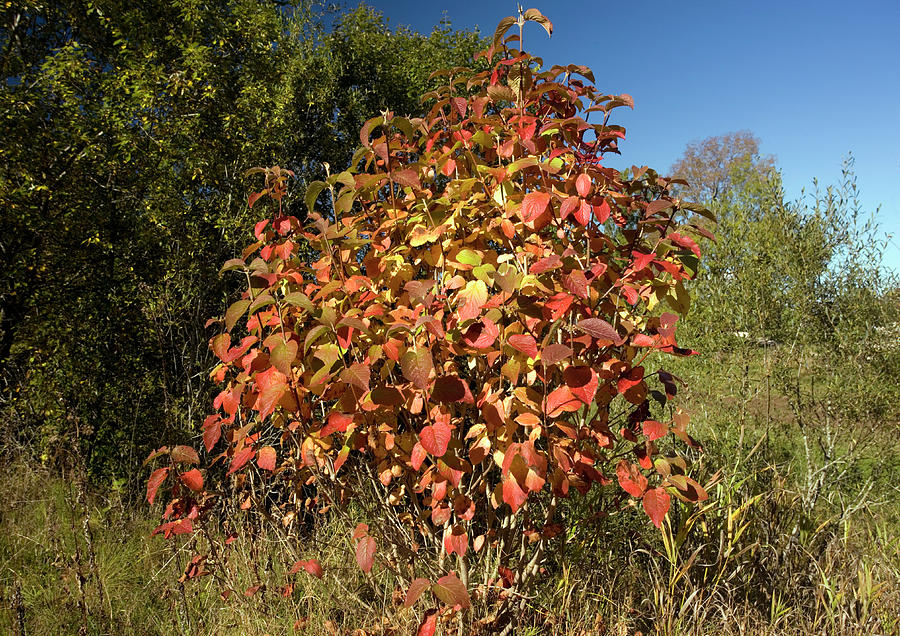The photograph captures an outdoor scene on a bright, sunny day, likely in the early autumn. Dominating the central part of the image is a large, bushy plant with vibrant leaves transitioning from red to yellow. This plant is not quite as tall as a typical tree but is larger than a regular bush. Below it, the ground is covered with long, light green to yellow grass, indicating that the area is not well-maintained. 

To the left in the background, there is a prominent tree with dark green leaves, while to the right, additional trees with green foliage can be seen. A clear, cloudless blue sky peeks through in the top right corner. The colors in the picture are vivid, with the red and orange hues of the central plant standing out sharply. The light and the clarity suggest the photo was taken in the middle of the day, with sunlight enhancing the brightness of the scene. In the far background, there is a hint of a structure, possibly a house, adding context to the natural setting.